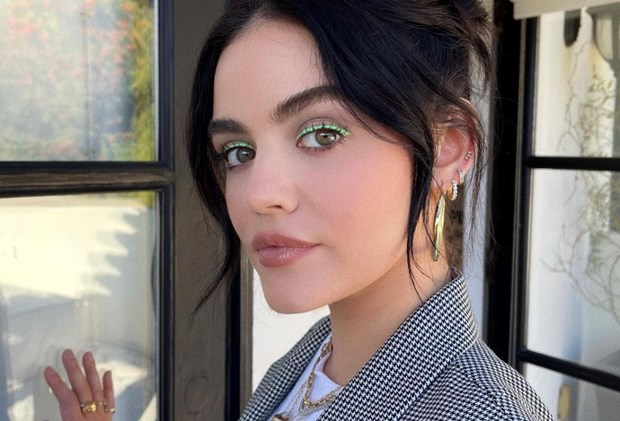A striking close-up image captures a poised woman standing near a glass-paneled door with brown trim. The woman, facing away from the viewer with her body oriented to the left, turns her head to gaze directly into the camera, exuding a subtle, almost serious expression. Her dark brown hair, tied back neatly, is softly accented by a couple of loose bangs framing her face. She sports vibrant green eyeliner that highlights her hazel eyes, complemented by carefully applied mascara, blush, and pink lip gloss. She is adorned with a large gold hoop earring, accompanied by smaller silver diamond hoops and studs in her right ear. In addition to her earrings, she wears several gold rings on the hand she has placed against the glass pane. Her attire consists of a black and white checkered blazer over a white t-shirt, highlighted by a couple of delicately layered gold necklaces. The background reveals an outdoor patio area, inferred from the reflections of trees and foliage through the window panes, adding an inviting natural element to the setting. The open glass door behind her reveals hints of a beautifully etched curtain, creating an intricate backdrop that frames her composed yet engaging presence.